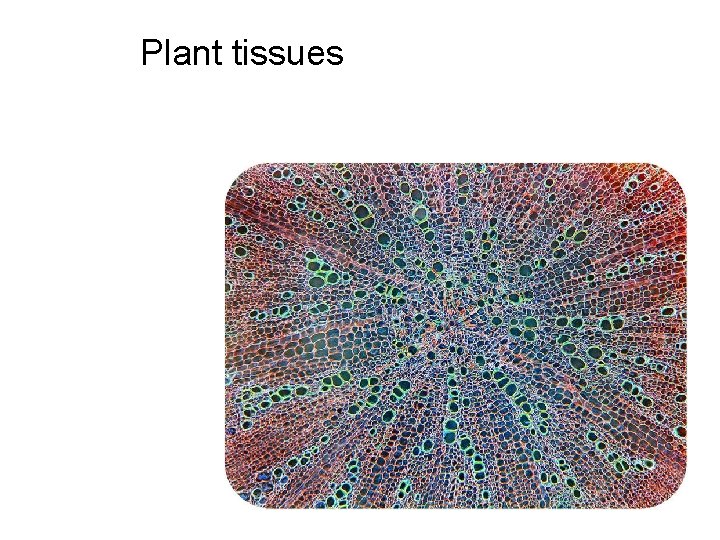The image features a white background with a smaller, postcard-sized section occupying approximately 45% of the total space, located in the bottom right corner. This section displays a highly detailed, multicolored microscopic view that resembles plant tissues, as indicated by black text reading "Plant Tissues" in the top left corner of the white background. The microscope view consists of numerous colored circular structures of varying sizes, predominantly green, which are the largest, along with white, red, blue, and purple circles. The green and dark green circles stand out significantly due to their larger size compared to the smaller red and blue circles. The circles are densely packed and create a three-dimensional effect, with colors blending from a brownish perimeter to blue and green toward the center. This gives the impression of looking into the bottom of a water well, where the different sized "cells" congregate and become more vibrant. The intricate pattern and diversity of colors merge in the middle, providing a striking and vivid composition.